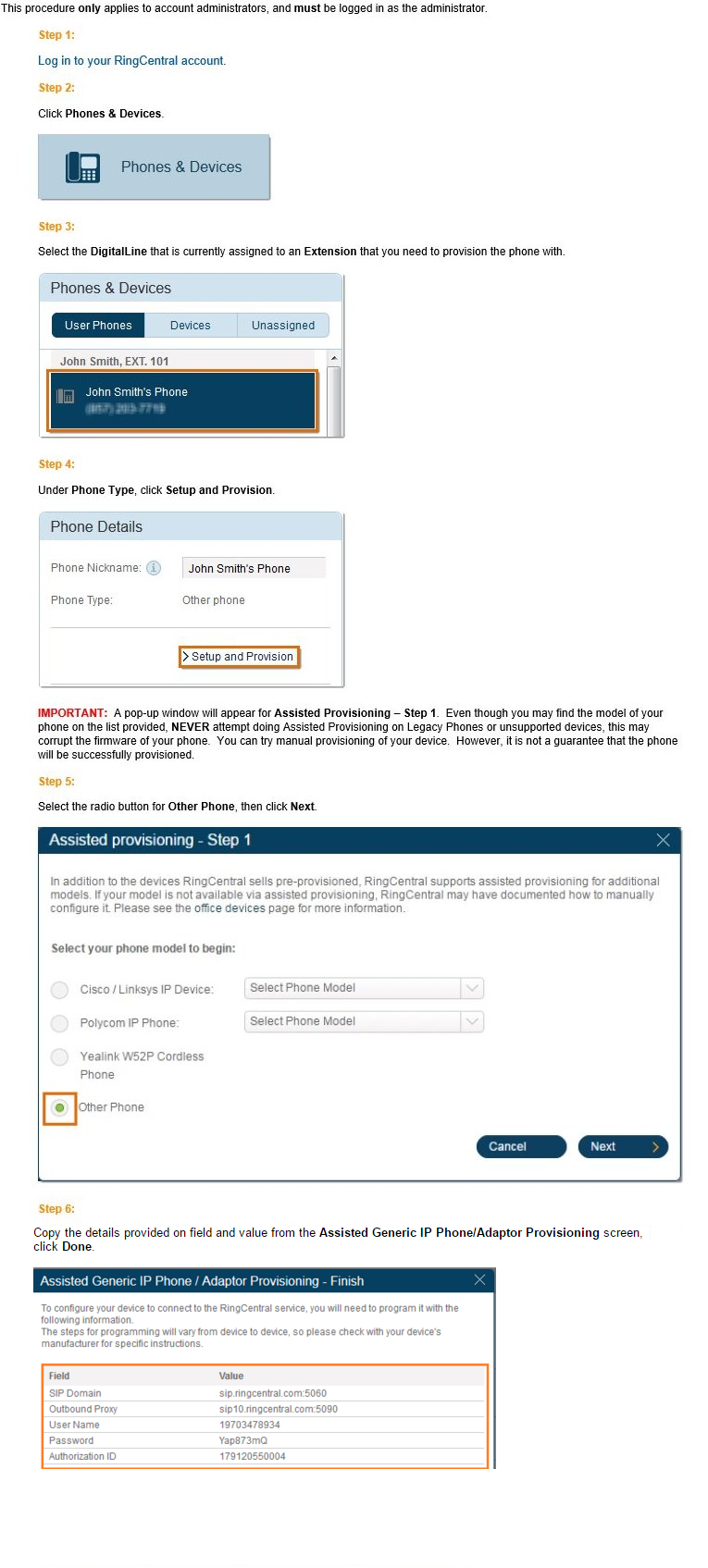**Step-by-Step Guide to Provisioning Phones in RingCentral for Administrators**

*This procedure is intended for account administrators and requires admin login.*

1. **Log into Your RingCentral Account**
   - Begin by logging into your RingCentral account as the administrator.

2. **Navigate to Phones and Devices**
   - Once logged in, click on the "Phones and Devices" tab as it appears within the interface. 

3. **Select the Digital Line**
   - Identify and select the digital line that is currently assigned to the extension you wish to provision the phone with. This will be under categories like "Phones and Devices," "User Phones," "Devices," and "Unassigned," displaying entries such as "John Smith's Phone."

4. **Setup and Provision the Phone**
   - Under the "Phone Types" section, click on "Setup and Provision." Here, you will view phone details before proceeding to the setup and provision stage.

5. **Important Note on Assisted Provisioning**
   - A pop-up window will appear for Assisted Provisioning (Step 1). Important: Although you may find the model of your phone on the list, **never attempt assisted provisioning on legacy phones or unsupported devices** as it may corrupt the phone’s firmware. It is recommended to attempt manual provisioning, though it is not guaranteed to be successful.

6. **Select "Other Phone"**
   - Choose the radio button for "Other Phone," then click "Next." The visual will show the selection for "Other Phone."

7. **Copy Information for Provisioning**
   - Copy the details provided in the "Field" and "Value" sections from the assistant generic IP phone adapter provisioning screen. Once done, click "Done" to complete the process.

*This guide ensures a smooth and correct provisioning of your RingCentral phones under administrative protocols.*